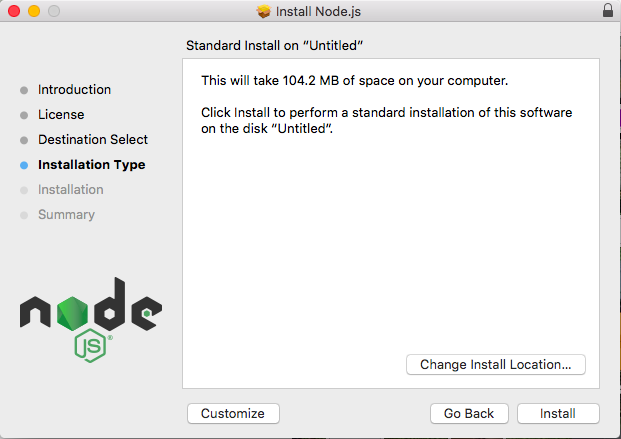### Detailed Caption

The image depicts an installation window for Node.js on a computer screen. The background of the window is gray. At the top of the window, there are three circles in red, yellow, and gray colors, respectively. Next to the gray circle, there is a red and yellow icon. The text "Install Node.js" is displayed prominently beside these elements. On the far right, there is an image of a locked padlock.

On the left side of the window, there is a series of navigational options displayed in a vertical column. These options are titled "Introduction," "License," "Destination Select," and "Installation Type," with "Installation Type" highlighted in bold black text. An aqua-colored button is also visible near this section.

Beneath this, the text states, "Standard install on Untitled." Below this line, a white box contains the additional information: "This will take 104.2 megabytes of space on your computer. Click install to perform a standard installation of the software on the disk Untitled."

Towards the bottom of the window, there is an option box labeled "Change Install Location." Additionally, three buttons are present: "Customize," "Go Back," and "Install." The target software is identified as Node.js, with "Node" displayed above and "JS" below.